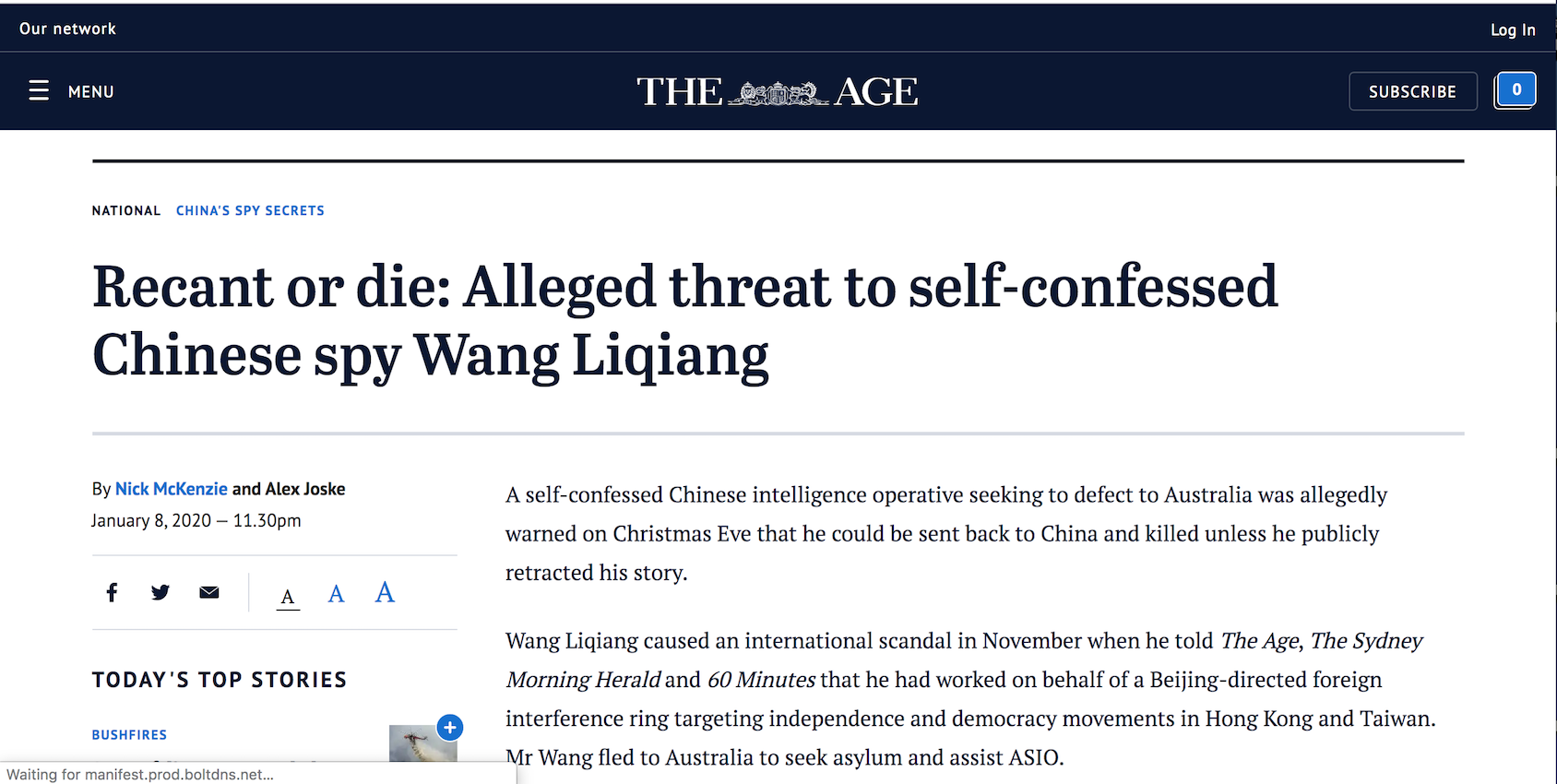This image is a screenshot of a news website. At the top, a navy blue banner stretches across the page. In the upper left corner of this banner, "Our Network" is displayed in white font, while in the upper right corner, "Login" is similarly positioned. Directly below this banner, centered on the page, the website's name, "The Age," appears in white font. A small, unidentifiable white icon is embedded within the middle of the word "Age."

To the right of the site's name, there is a "Subscribe" button, and to the left, a "Menu" button. Beneath this header, the main body of the webpage is a stark white, featuring an article.

The headline of the article reads, "Recant or Die: Alleged Threat to Self-Confessed Chinese Spy Wang Likwang," authored by Nick McKenzie and Alex Joske. The publication date and time, January 8, 2020, at 11:30 PM, are listed immediately below the headline.

Situated near the headline are sharing icons for Facebook, Twitter, and YouTube. Additionally, there is a font size adjustment option featuring three blue "A" icons, signifying small, medium, and large text sizes. The small "A" is currently selected.

Further down the page, a section labeled "Today's Top Stories" precedes the main text of the article.